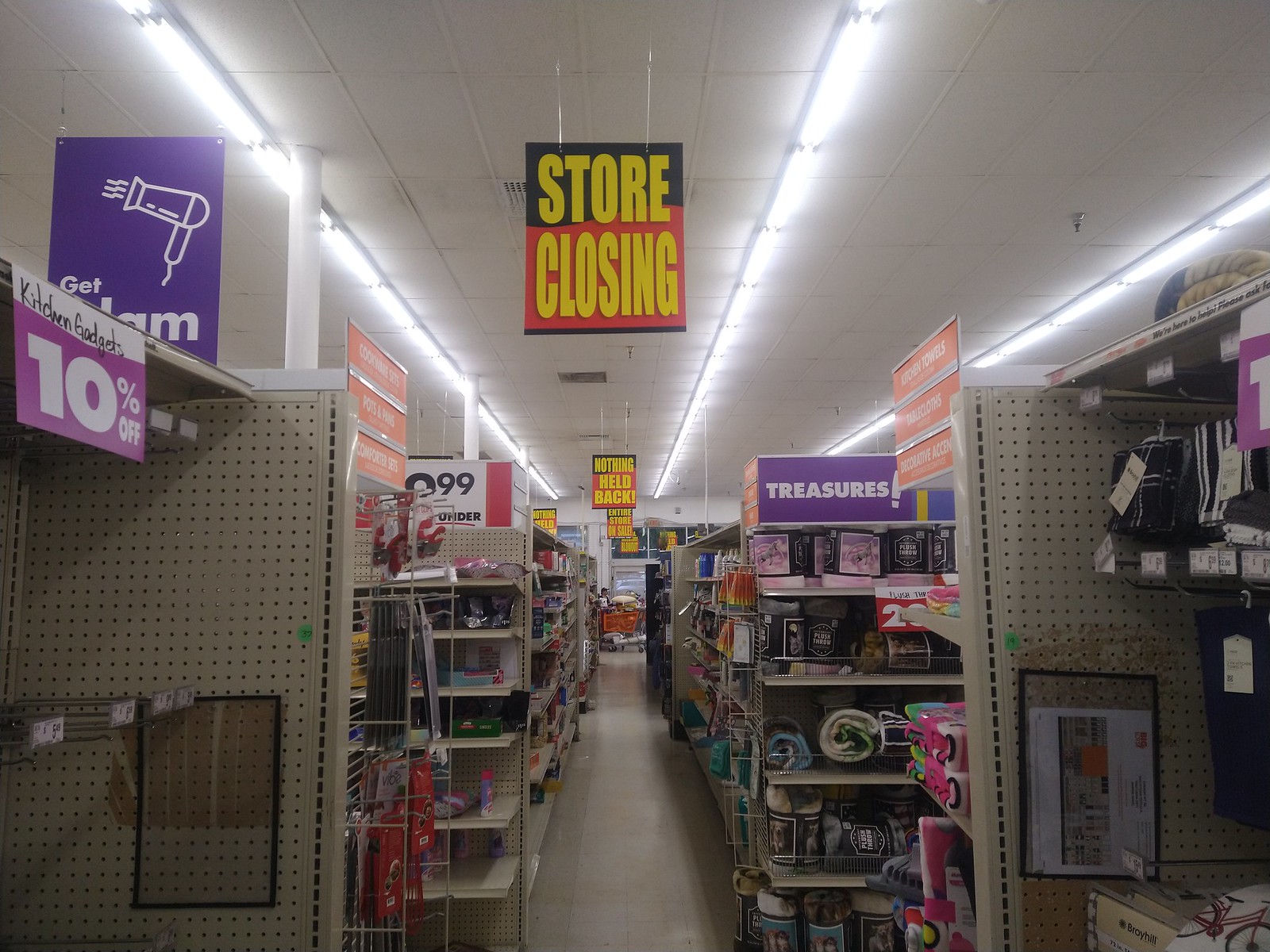This color photograph captures the interior of a large department store undergoing a going-out-of-business sale. The image features a central aisle lined with various shelves and racks on both sides, leading to the far end of the store. Dominating the scene are numerous signs hanging from the drop ceiling, the most prominent being one in the foreground that reads "Store Closing" in large, bold yellow letters on a black and red background. Similar signs with phrases like "Nothing Held Back" are visible throughout the store.

The aisles are sparsely populated with items, emphasizing the clearance nature of the sale. A rack labeled "Kitchen Gadgets" with a handwritten "10% off" sign stands empty, while another side displays dishcloths also marked down by 10%. Some end caps feature signs like "Treasures!"—highlighting an assortment of small portable heaters and throw blankets at a 20% discount. A nearby purple sign with a white hair dryer reads "Get Glam."

Additional details include fluorescent lighting overhead and a tan-to-off-white floor below. The shelves hold a random assortment of household items such as blankets, towels, and bottles of cleaning products or shampoo. In the distant background, there is an unattended orange shopping cart, adding to the sense of a store winding down its operations.